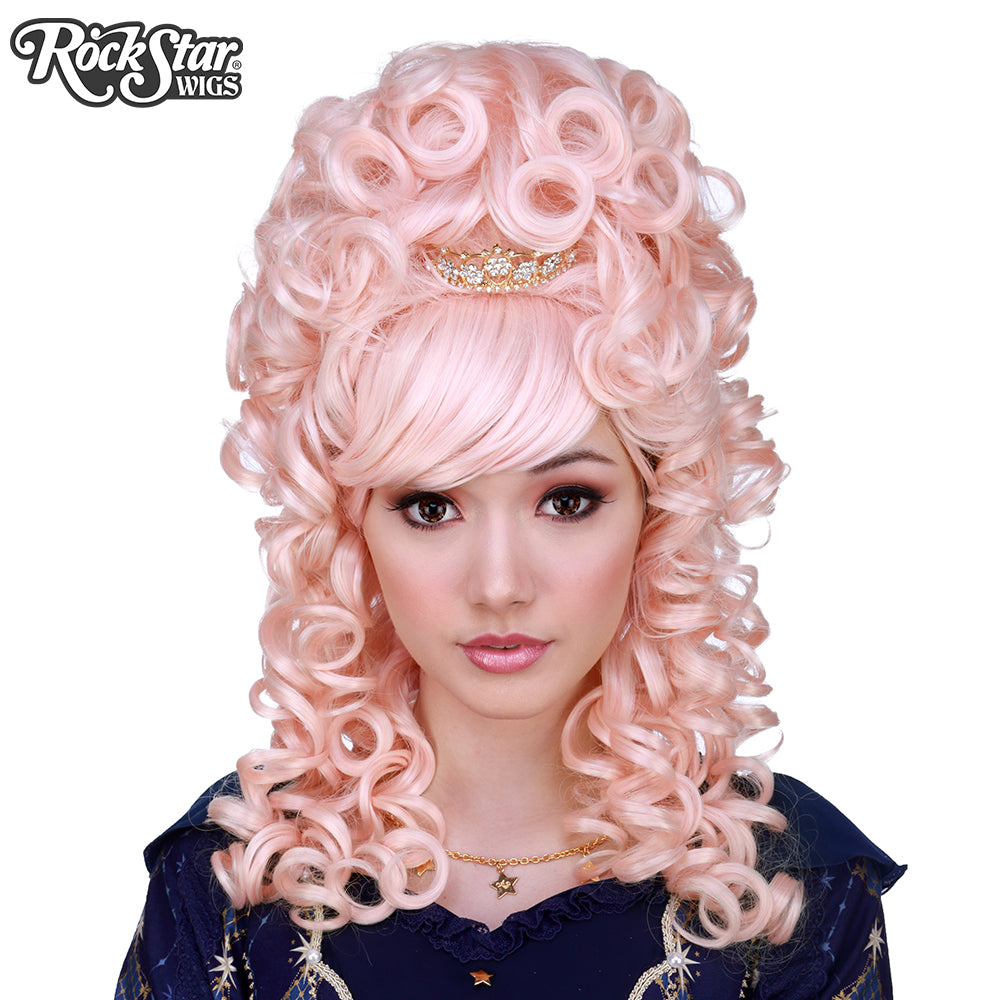This image captures a young Caucasian woman with a strikingly voluminous pink wig, styled in Dolly Parton-esque bouffant curls cascading past her shoulders. Nestled in the wig's carefully crafted curls is a diamond-studded tiara, enhancing the whimsical look. The wig also features a section of curly bangs. The woman’s makeup is meticulously applied, with pink lipstick matching her wig, black mascara accentuating her eyes, and a touch of blush highlighting her cheeks. Her large brown eyes lend to her bright and engaging expression, as she gazes directly at the viewer with her mouth slightly open, revealing a peek of her two front teeth. She wears a navy blue top adorned with tiny white shooting stars and red accents, just beneath which is a gold necklace with a gold star pendant. The top button of her shirt is also gold, framed by small pearls on either side. The background is a plain white, and in the upper corner of the image, there is a logo that reads "Rockstar Wigs."